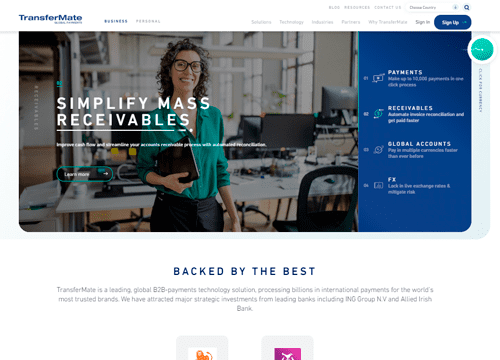The TransferMate website, a leading global B2B payments technology solution, features a neatly arranged layout with the company's name prominently displayed in the upper left-hand corner. The "TransferMate" logo, in blue with a capital 'T' and 'M' and no spaces between the words, is clearly visible. To the right of the logo, visitors can toggle between 'Business' and 'Personal' options; 'Business' is currently highlighted in blue, while 'Personal' appears in gray.

Further to the right, users can select their country of operation and access links to the blog, resources, or contact us pages. A blue "Sign Up" button with white text invites new users to register.

The main section of the homepage showcases a professional image of a woman in an office setting. She is dressed in black pants and a green long-sleeve shirt with the sleeves rolled up to her elbows. In her right hand, she holds what appears to be either a black book or a small laptop. Her left arm hangs naturally by her side. This woman, adorned with glasses, has shoulder-length, moderately curly hair and is of Caucasian descent.

The background displays a typical office environment with tables, computers, and chairs. Overlaying this image, in bold white capital letters, are the words "SIMPLIFY MASS RECEIVABLES."